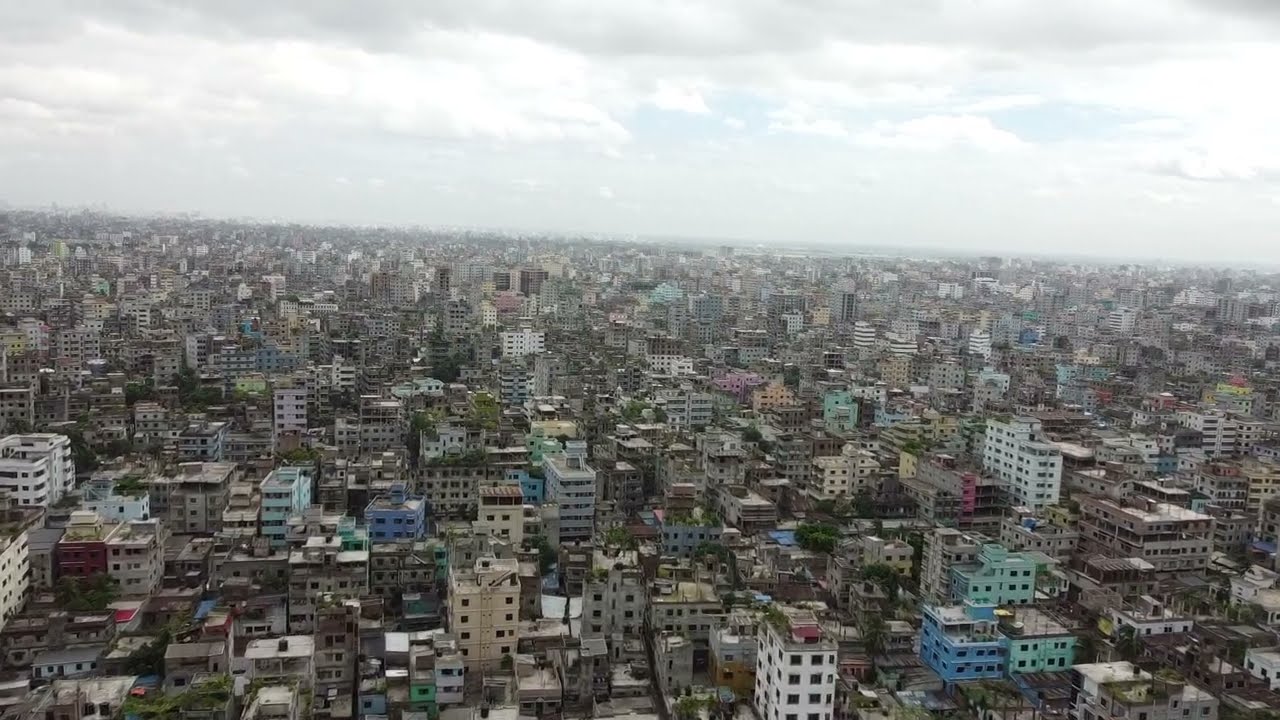This aerial photograph, likely captured by a drone or from a helicopter, reveals a vast, densely populated shanty-style city that bears resemblance to South American or perhaps Brazilian urban landscapes. The shot was taken during the daytime, with the upper third of the frame showcasing a sky filled with a mixture of white and grayish clouds, contributing to a subtle smoggy haze, though patches of blue sky peek through. The bottom two-thirds of the image are dominated by a sprawling array of buildings, none exceeding ten stories in height. These structures are closely packed together and exhibit a vibrant palette of whites, blues, greens, browns, and reds. The buildings, which appear to be mainly apartments, share a similar design featuring dark window frames. Sprinkled intermittently among the buildings are small clusters of trees. The overall impression is of an older, colorful city bustling with architectural uniformity and teeming with life.